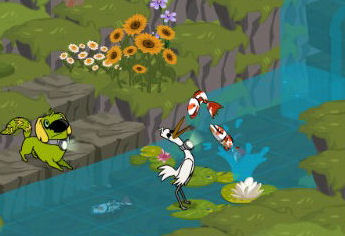The image appears to be a screenshot from a cartoon. It depicts a tranquil water scene filled with green lily pads. Positioned prominently on one of the lily pads is a white stork, wearing sunglasses. Around his neck hangs a small, illuminated flashlight, pointed upwards. The stork gazes upward, seemingly preparing to catch fish leaping out of the water.

To the right of the scene, a grassy cliffside rises sharply from the water's edge. Further back, additional cliffs can be seen, some adorned with grass and colorful flowers. Another character stands on the edge of a nearby cliff: a green dog with yellow ears and a black nose. Like the stork, the dog also wears a flashlight around its neck, although this flashlight is directed towards the stork.

The entire scene is vibrant and dynamic, emphasizing the anticipation and interaction between the cartoon characters.